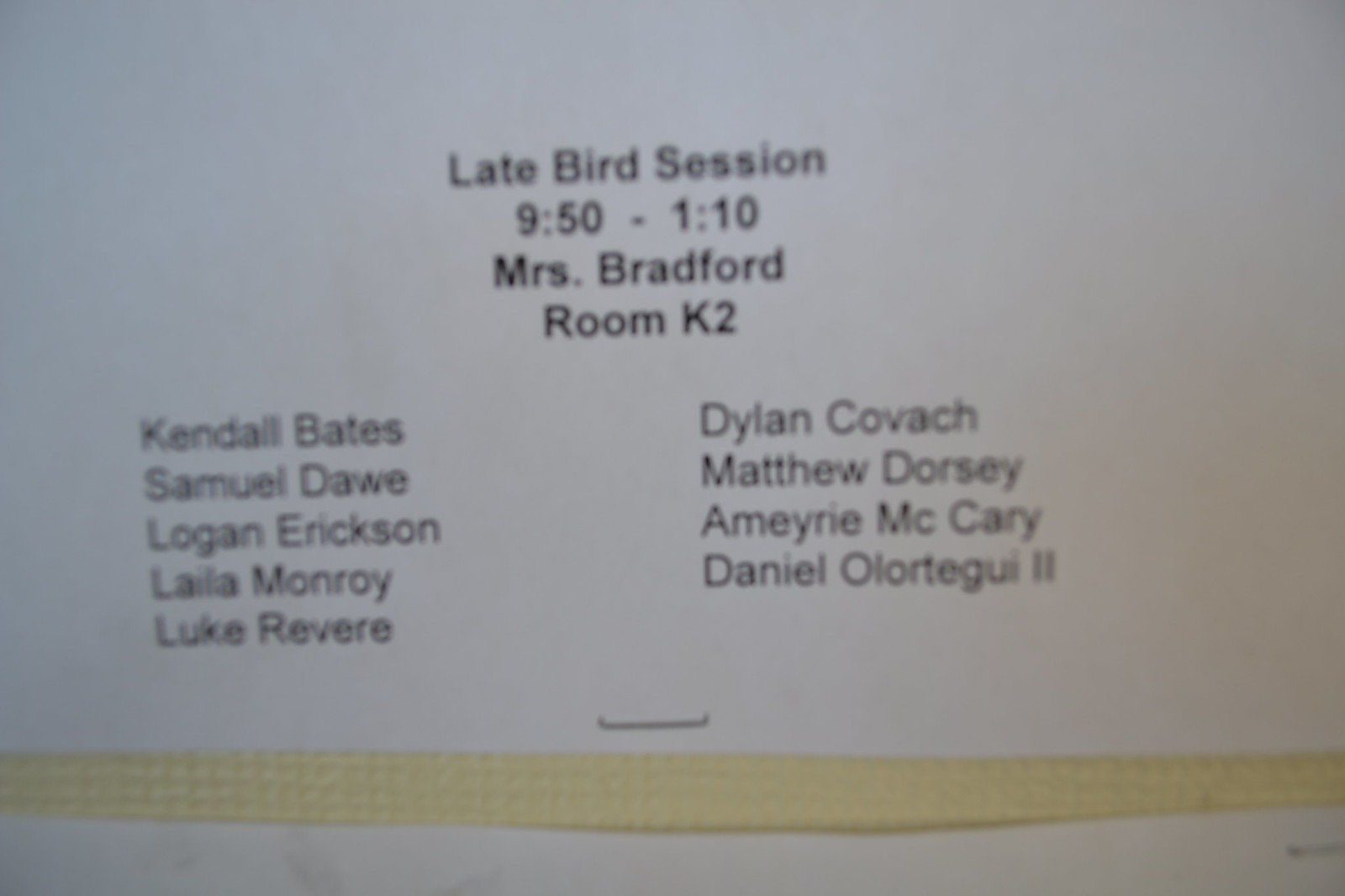The image is an out-of-focus photograph of a printed document on a white background. At the top center, in bold black text, it reads "Latebird Session, 9:50-1:10". Below this, it says "Mrs. Bradford" followed by "Room K2". There are two columns of names below this information; the left column lists Kendall Bates, Samuel Dahl, Logan Erickson, Lela Monroe, and Luke Revere, while the right column includes Dylan Kovach, Matthew Dorsey, Amiri McCarry, and Daniel Olortegui II. A noticeable feature of the document is a yellow ribbon-like stripe running horizontally across the middle. The paper appears slightly blurry but still legible, with staples present near the middle and the lower right corner.